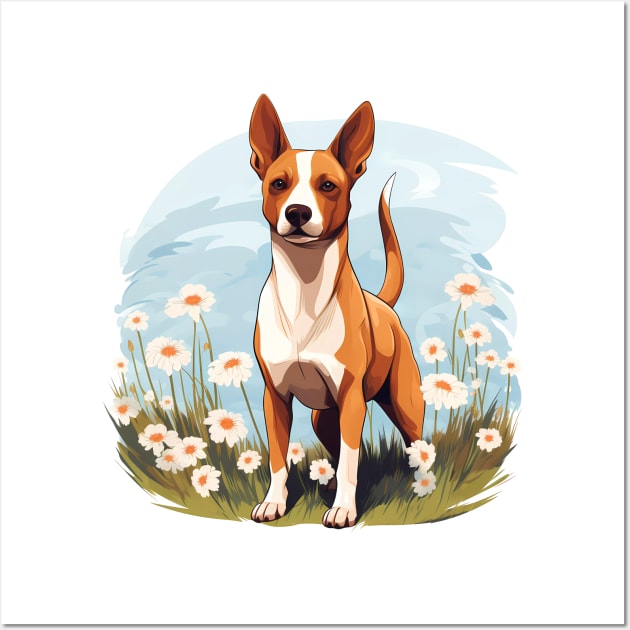This image features a highly detailed, hand-drawn depiction of a dog, possibly a beagle, characterized by its tall ears and distinctive brown and white coloring. The dog's fur is predominantly brown on its back, sides, and the top of its head, while the underbody and the center of its face are white. Additional white patches are present on its front paws, and its tail has a white tip. The dog stands in a field of green grass, surrounded by white flowers with pink or yellow centers. The background showcases a sky-blue color with a subtle bubble effect, enhancing the depth and contrast of the scene. The overall style combines elements of hyper-realism and pastel illustrations, providing a vibrant and life-like but slightly cartoonish appearance. The artist's use of illustrated software is evident in the stylized portrayal, adding a modern, digital touch to the hand-drawn aesthetic. The dog is centrally positioned, standing at attention as if ready to play, with a bright and lively expression in its brown eyes, making it the clear focal point of this visually striking artwork.